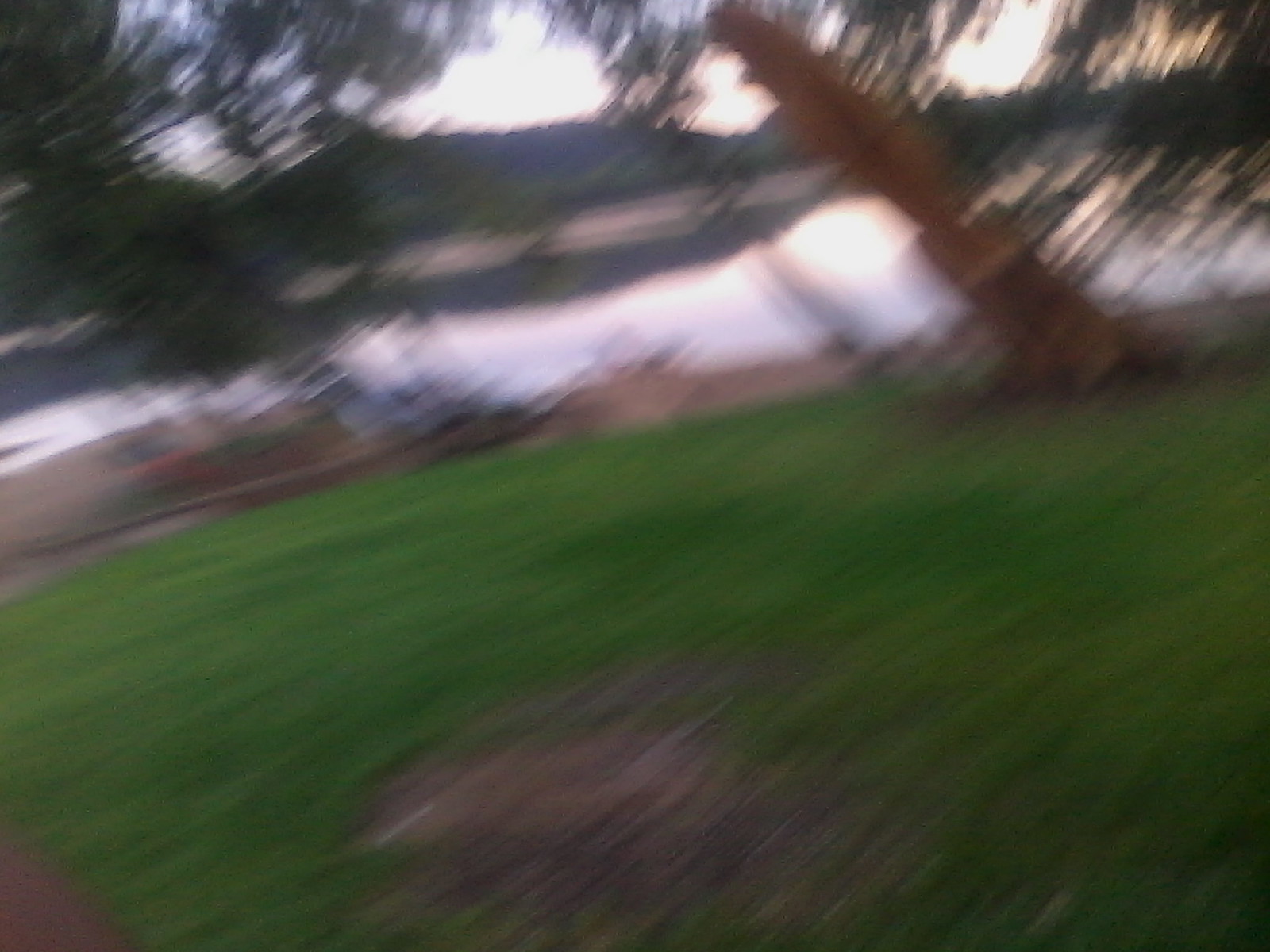This outdoor photograph, likely taken while in motion, is very blurry with the streaks suggesting side-to-side movement. In the foreground, there is a lot of green grass with a small dirt or mud patch peeking through. Beyond the grass, there's a thin, brown strip that could be a beach or shoreline. This transitions into a body of water, possibly a lake, which reflects the sky above with a hint of the sun towards the horizon, indicative of dusk. The background features some hills or dark mountains, although the blur makes it difficult to distinguish. The photo is taken at a slight angle, adding to the motion effect, making the scene appear less distinct.